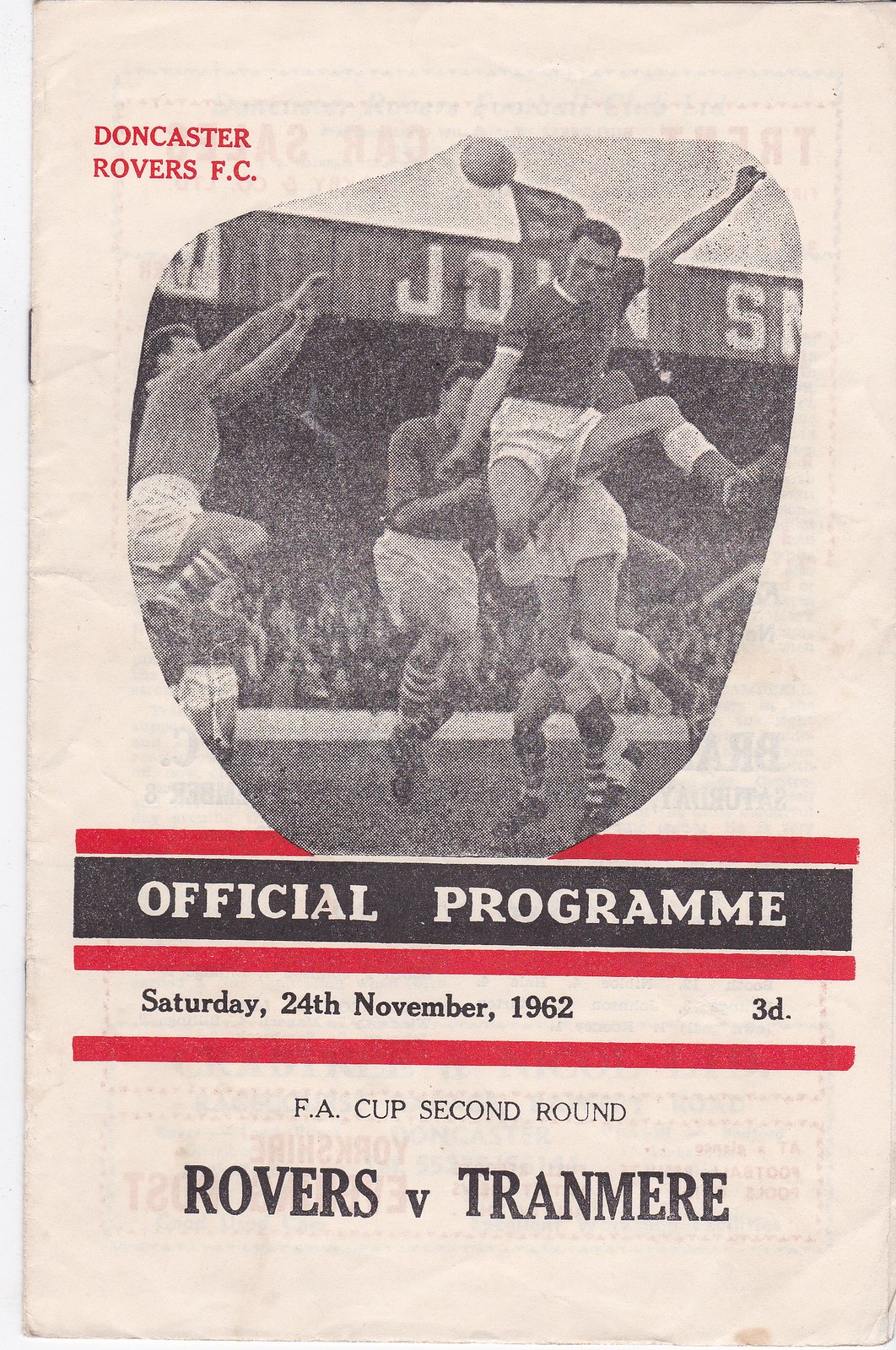This color photograph showcases the front cover of a vintage sports program from the Doncaster Rovers Football Club. It's printed on pink stock with a central, somewhat grainy black-and-white photograph depicting about six young men in mid-air actions, suggesting a lively soccer game. Dominating the top left corner is the text "Doncaster Rovers FC." Directly beneath the photo, bold, white capital letters within a black banner, framed by a red border, proclaim "Official Program." Further down, similarly bordered text details the event: "Saturday, 24th November, 1962, 3D," indicating the date and price. Near the bottom, another bold statement reads "FA Cup, Second Round," with "Rovers vs. Tranmere" prominently displayed, informing the reader of the competing teams. The overall design, the varied colors (tan, red, gray, black, white), and the position of the elements suggest this is a nostalgic piece one might have received at the entrance of a live soccer match.